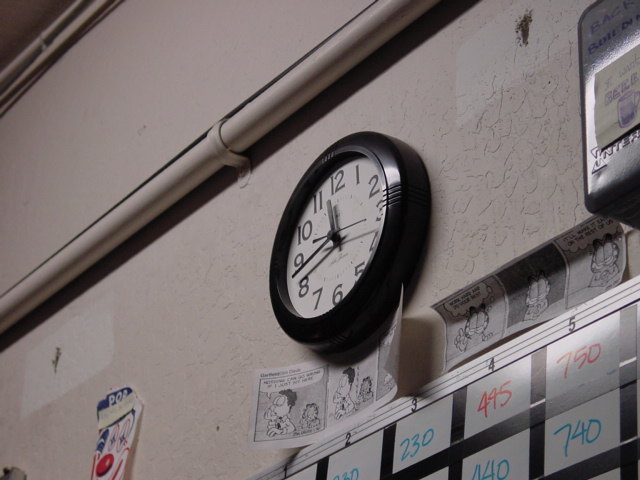This photograph, shot from below at an angle looking up to the left, captures a detailed corner of a white wall. Dominating the scene is a black plastic-framed round analog clock displaying the time at approximately 11:42, with the second hand just past the three. Above the clock, a white pipe runs horizontally across the wall, secured with a U-bracket. The pipe extends through the entire image from left to right.

Directly below the clock, two black and white Garfield comic strips are pinned to the wall, their edges slightly curved, suggesting they are not fully taped down. Adjacent to the comics, appears a metal-framed board covered with white placards or possibly a grease board, displaying a grid of numbers drawn in marker; these include 232, 445, 750, 440, and 740. Some of the numbers are red and some blue, organized into columns numbered 1 through 5 at the top. 

The image also captures an area of miscolored concrete with visible holes and a hasty patch paint job above the clock. Above the numeric grid, a set of cut-out Garfield cartoons can be seen, fitting neatly below the clock. In the top right corner, there is a metal box, possibly an industrial device or electronic equipment, with an unreadable label affixed, giving a functional ambiance to the scene. This richly detailed snapshot invites a closer look into the eclectic mix of orderly information and casual decor on this particular wall.